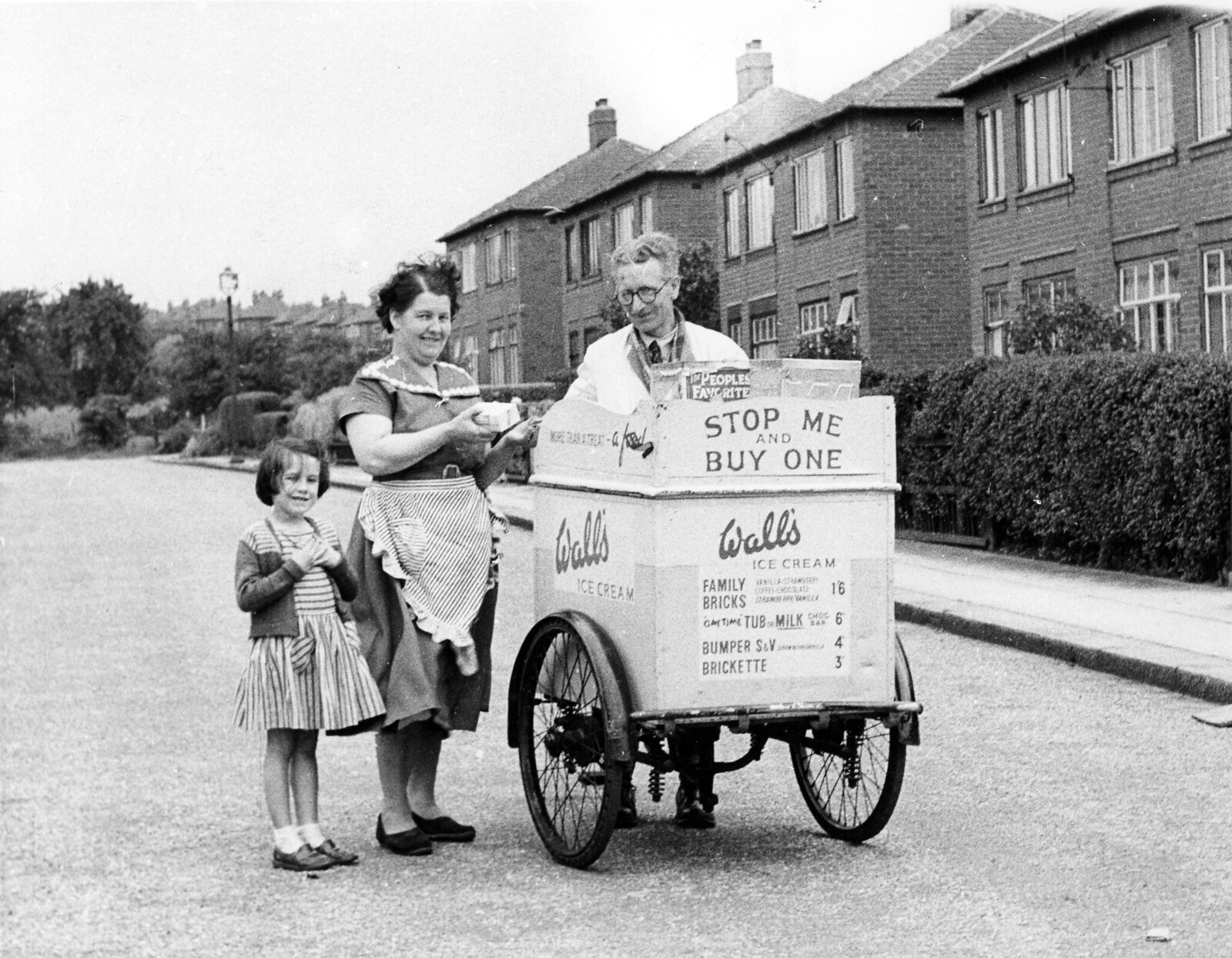In this black and white photograph, a man, woman, and little girl are positioned on a clean, ascending street lined with brick row houses and hedges. The street curves left and up, away from the viewer. On the right side of the street is a sidewalk that runs in front of the brick buildings, topped by trees in the background. In the center of the photo stands an ice cream vendor behind a classic two-wheeled cart. The man, with medium-length hair and eyeglasses, wears a white coat over a plaid shirt, visible mostly from the shoulders up as he stands behind his cart. Prominently displayed on the front of the cart is the text "Stop Me and Buy One," followed by "Walls Ice Cream" and a menu listing several choices with prices. The cart, facing slightly to the right, also features a Walls sign on its left side and has large spoke wheels. To the left of the cart, a woman with short dark hair is wearing a dress and a white apron, smiling and holding an ice cream. Beside her stands a little girl with dark hair in a striped dress and sweater, both gazing slightly to the right.